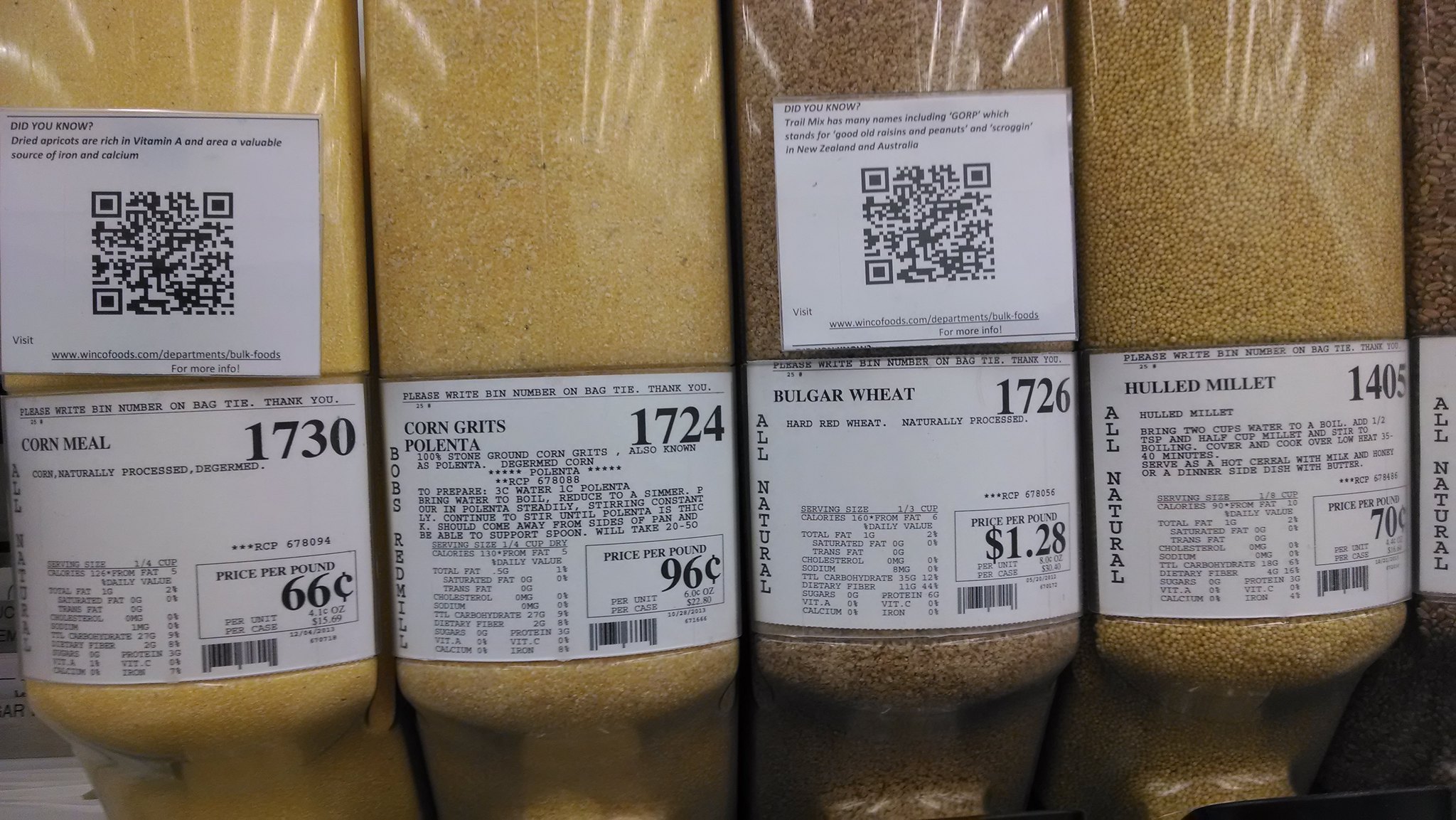This photograph, taken inside a store, features a display of various grains packaged in clear plastic jugs, each with identifiable tags and barcodes. Starting from the right, the first jug contains millet, labeled with the number 1405, priced at 70 cents, and designed to be easily poured out. The next jug holds bulgur wheat, marked with the number 1726 and a barcode, priced at $1.28. This grain is darker brown in color. To its left, there is a jug of corn grits polenta, a golden grain, labeled number 1704. The final jug on the left contains cornmeal, also golden but slightly more vivid than the polenta, with the number 1730 and a barcode, priced at 99 cents. Each jug features stickers providing details such as the product name, code, price, and some nutritional and allergy information. The display is likely part of a self-service bulk section where customers bring their own containers for shopping. Reflections of store strip lights can be seen on the surfaces of the plastic containers, adding to the detailed clarity of the image.